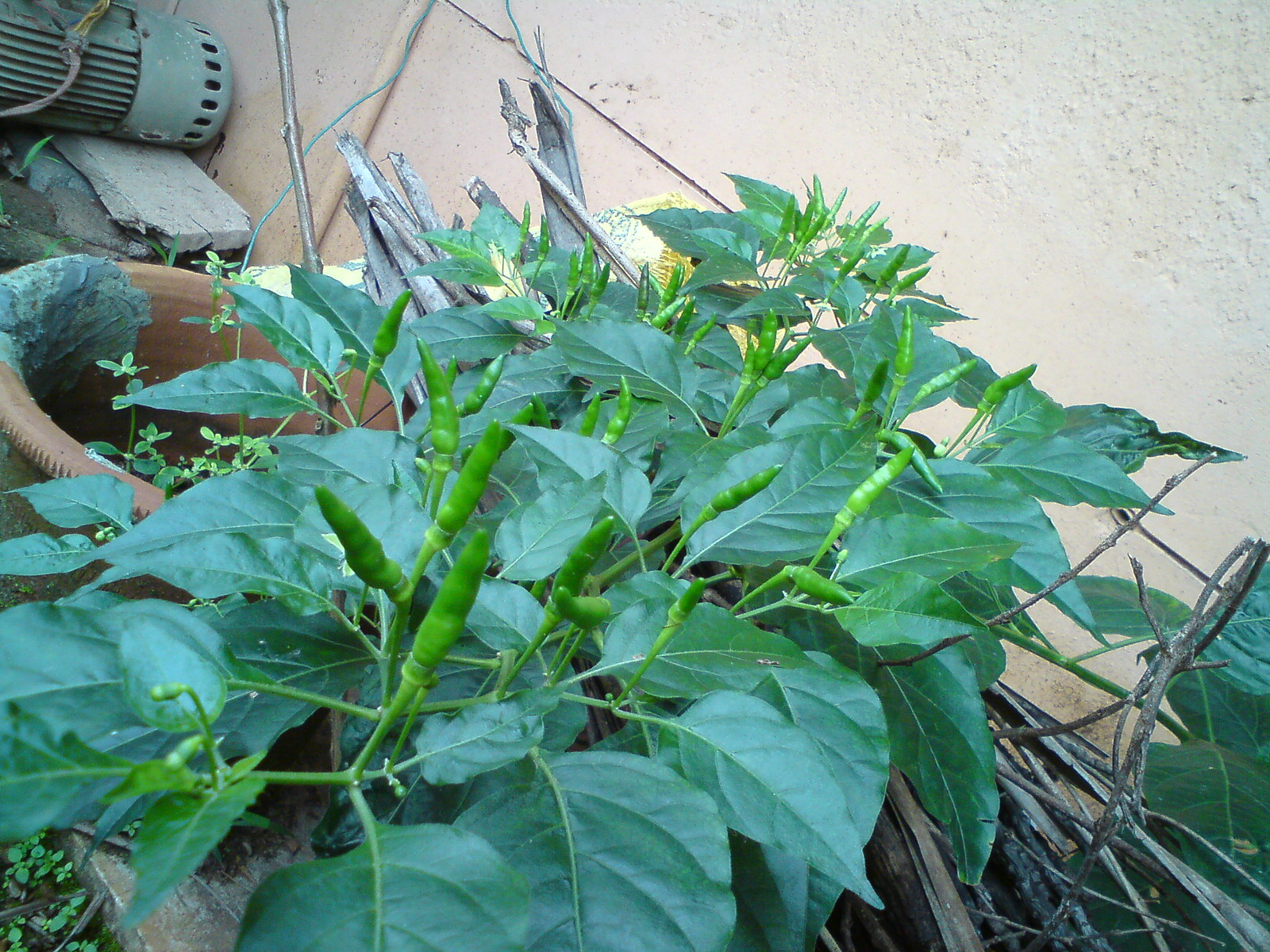This detailed photograph depicts a vibrant pepper plant growing outside against a beige stucco wall. The plant, which boasts broad, pointed green leaves with bluish undertones, is situated in a backyard garden setting. The peppers are long, thin, and grow upright from the stems, characterized by their bright green color with yellow undertones and slightly lobed, bumpy texture. In the upper left-hand corner of the image, an old gray motor, encircled by a dingy strap and resting on a cracked wooden board, adds a rustic element. The background reveals additional details, including a brown flower pot with some green clover-like plants along its edge, and scattered dead twigs intertwined with other debris.